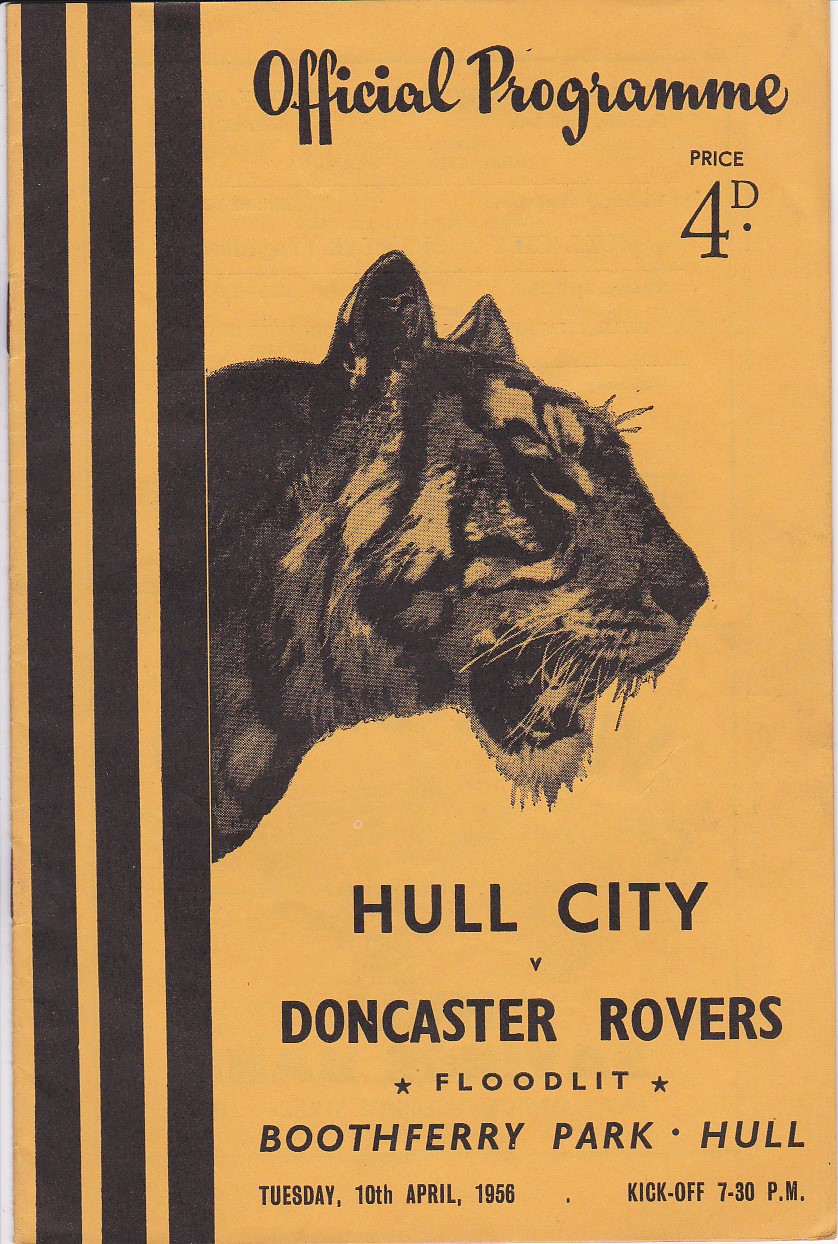This is a vintage, rectangular soccer program cover from April 10, 1956. Its predominantly yellowish-gold background is accented with three thick, vertical black lines running down the left margin. At the top, in an elegant calligraphy font, it reads "Official Programme". Below this, on the right, the price is marked "4D". Dominating the center of the cover is a captivating black-and-white drawing of a roaring tiger, shown in side view with distinctive stripes and a black nose. Below the tiger, the program details are presented in black text: "Hull City," followed by "v. Doncaster Rovers," "Floodlit," "Boothferry Park, Hull," "Tuesday, 10th April, 1956," and "Kick-off 7.30 PM". The booklet is small and stapled with two staples for binding, combining striking visuals with comprehensive match details.